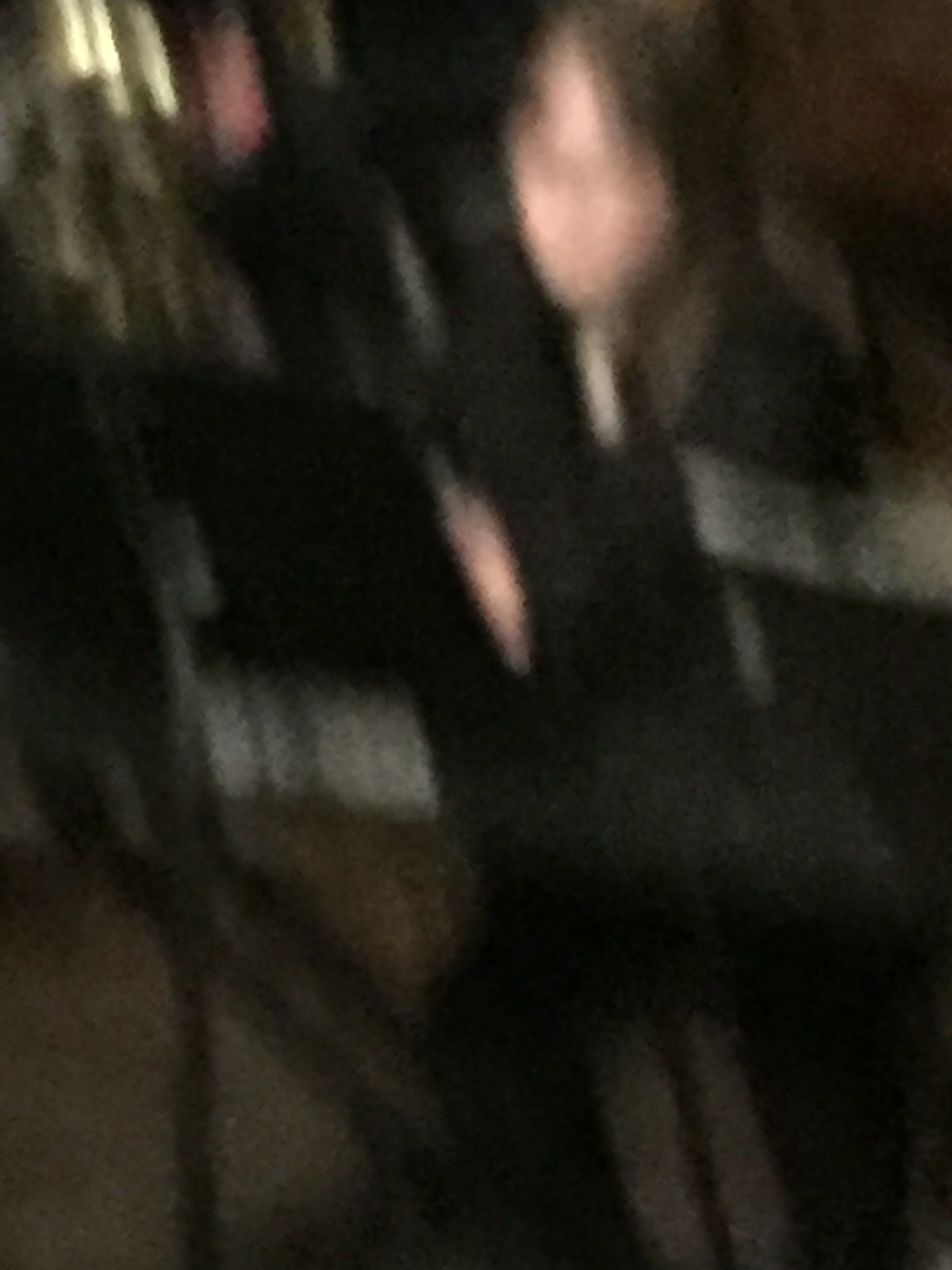This image is a vertical color photograph characterized by significant blurriness and graininess, giving it an abstract, painterly quality. The scene appears as though viewed through frosted or bumpy glass, with an impressionistic feel. At the center-left of the image, there is a discernible figure, possibly a girl, leaning towards the left, with her feet extending to the bottom right. To the left of the figure stands what seems to be a music stand holding a book, suggesting she might be reaching or leaning towards it. The photograph features a muted color palette dominated by dark black, medium gray, and orangish-yellow hues, interspersed with flesh tones and streaking effects. In the top left corner, three yellow lines stand out against the background. Overall, the obscure artistic style of the photograph suggests it may have been captured using specialized filters or techniques to enhance its streaked and abstract appearance.